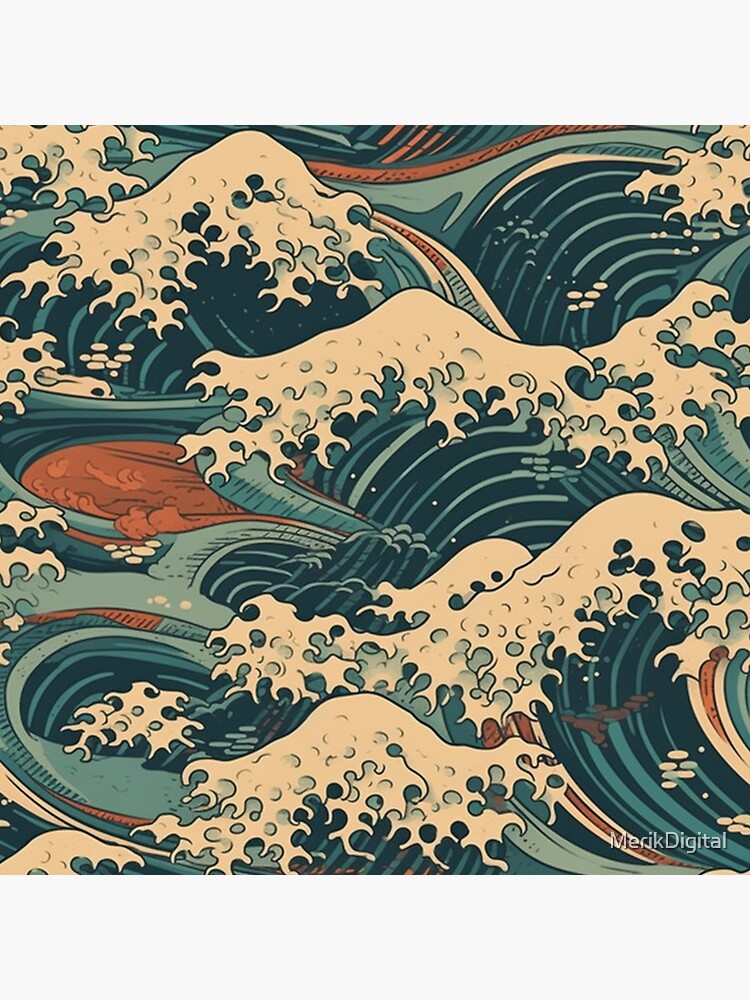The image is a detailed digital illustration rendered in the style of traditional Japanese art, reminiscent of "The Great Wave off Kanagawa." It features an intricate pattern of ocean waves in dark blue, light blue, aquamarine, and green, topped with white foam. The waves are consistently portrayed across the artwork, forming a repeating pattern that could be suited for wallpaper or textile design. Occasional red swirling water and touches of brown add an abstract element to the piece. The artwork is signed in the bottom right corner with a watermark that reads "Merrick Digital." The overall appearance is of a stormy sea with a harmonious blend of colors creating a visually captivating and richly detailed scene.